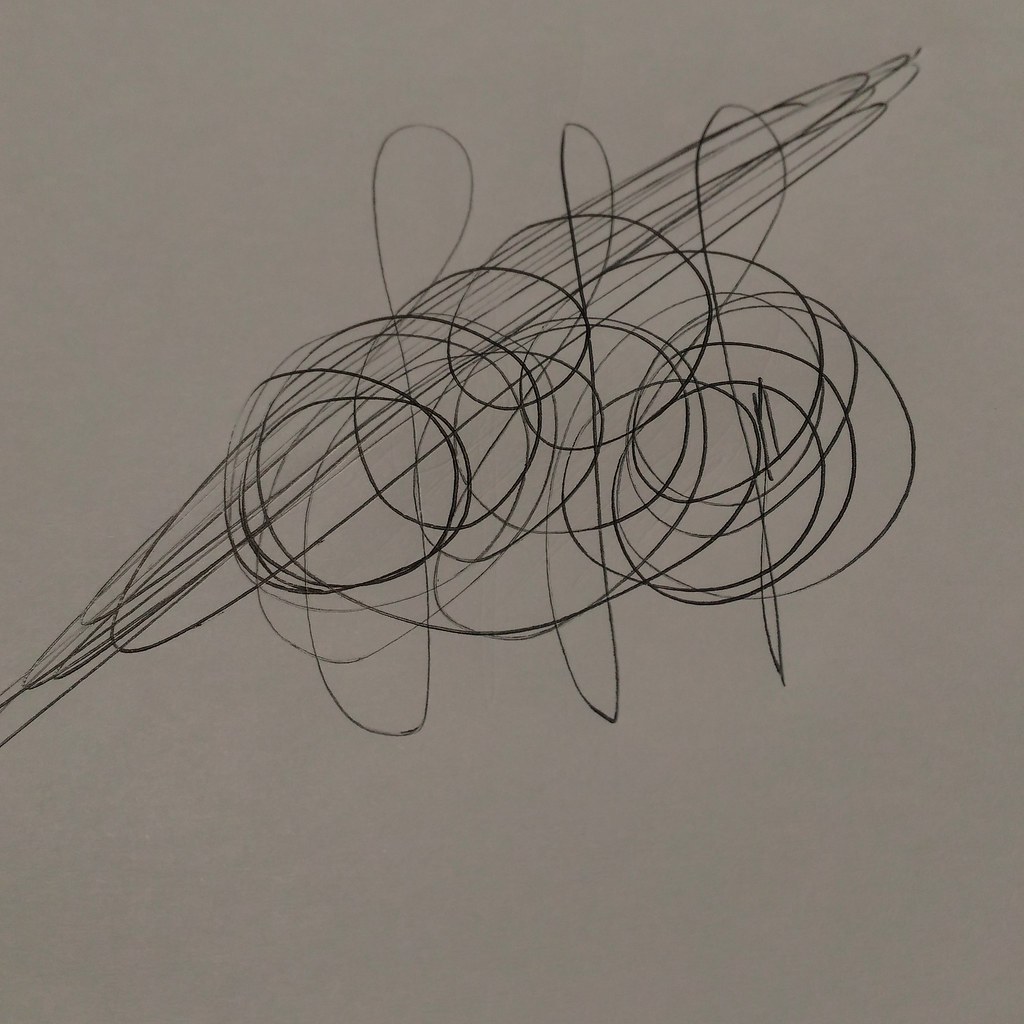An indoor color photograph captured from above depicts a sketchpad sheet oriented vertically. Dominating the center of the page is a doodle executed in dark black ink or pencil. The background design features a series of overlapping, elongated ovals, approximately seven to eight in number, originating near the lower half of the left edge and extending towards the upper right corner.

In the central area, the artist appears to have attempted drawing a cursive letter "J" three times—one centrally located and the others flanking it to the right and left. Over these initial attempts are 10 to 15 circular loops, overlapping and intertwined, creating a densely packed abstract form resembling a blob.

The overall image is monochromatic, with no colors, words, text, or printing visible. The photograph is somewhat dark, but the focus remains sharp, clearly showing the crisp and dark lines. Notably, there is no signature at the bottom, suggesting this is not a piece of finished artwork but rather a page filled with spontaneous practice doodles, possibly reflecting a moment of frustration. The corners of the sketchpad, particularly the upper left and right, are devoid of any drawings. The pressure applied by the artist is evident in the boldness and clarity of the lines, indicating a firm grip on the pen or pencil.